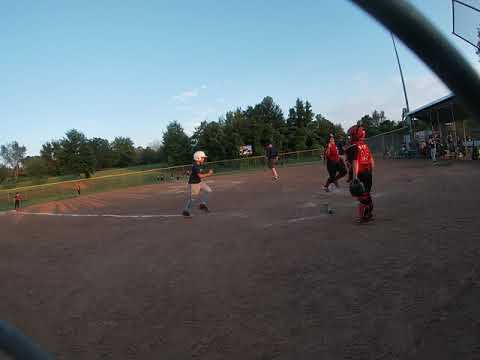This image captures a lively little league baseball game from the perspective of home plate, taken right behind the backstop. The field is primarily bare dirt featuring faint, blurry white baselines. The diamond and the kids playing are shadowed, while the grass in the outfield and the trees behind are bathed in sunlight. A young boy, likely around eight or nine years old, wearing a black shirt and a white helmet, is sprinting from third base to home plate. 

Adjacent to the field, a modest white fence encloses the area on the left and somewhat on the right, which is also flanked by a building where several children are gathered. 

One team is dressed in black shirts with white helmets and khaki pants, while the other team sports red shirts, red helmets, and black pants. The boy attempting to score is in the uniform of the black-shirted team. Coaches or adults can be seen, likely providing supervision, particularly near the center-right of the pitch areas. Additionally, there are clusters of people at various bases, including a noticeable group near second base. 

Beyond the playing field, the background descends into a scenic hillside dotted with trees, where spectators are seated, enjoying the game. Both teams’ dugouts are visible on the right side of the photo, populated by players and other kids watching the game unfold.